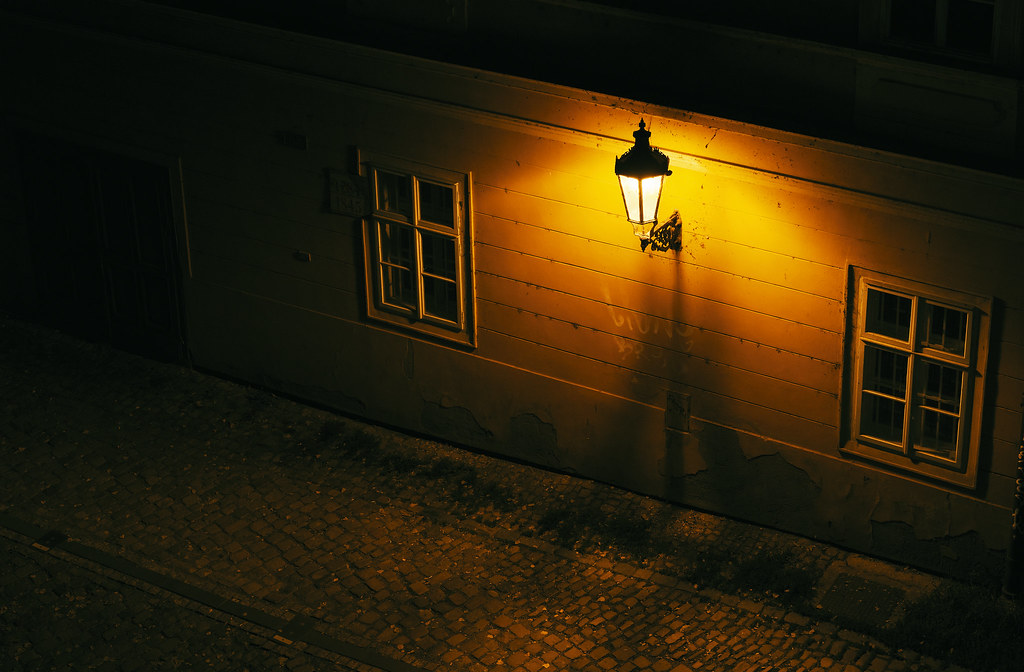The image captures a nighttime scene of an exterior wall of a house, illuminated by a striking golden lamp. The lamp, which has a black metal top and glass surrounding the bulb, is mounted centrally on the wall and serves as the primary light source, casting a bright, eerie glow across its surroundings. The house's wall features long horizontal wooden panels, and beneath the lamp, there are faint, smudged markings that appear to be illegible graffiti.

On either side of the lamp are two rectangular windows, each divided into six square panes of glass. The darkness obscures any view inside, but there's a hint of bars behind the window on the right side. The ground below is a sidewalk composed of variously sized cobblestones and bricks, giving a textured, rough appearance. The entire environment beyond the reach of the lamp's light fades into pitch black, contributing to the sense of eerie desolation.